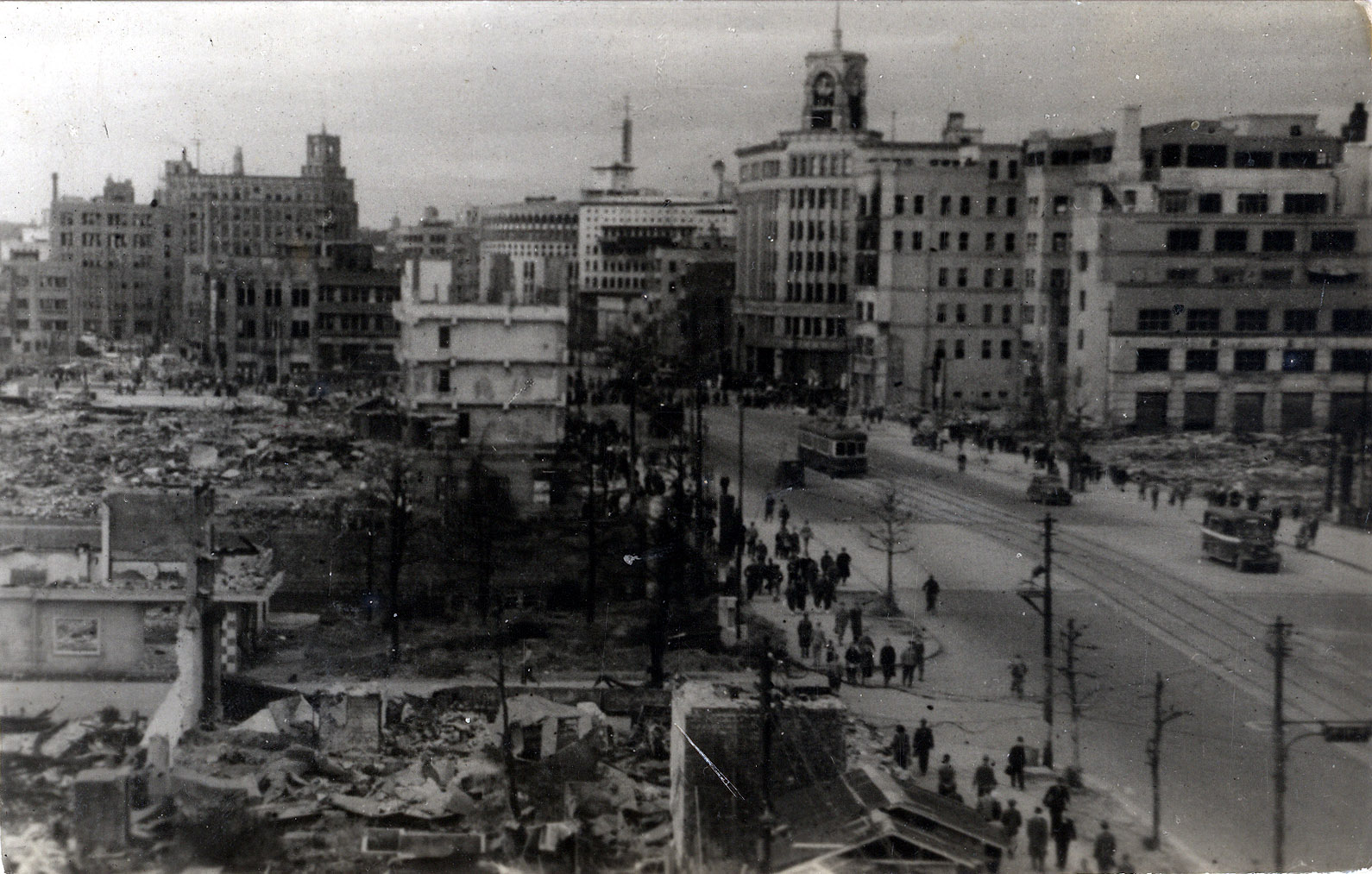The black and white photograph captures a cityscape from the early to mid-20th century, likely post-event owing to the visible destruction. Dominating the background, a series of multi-story buildings extend horizontally from the left to right edge. In stark contrast, the foreground on the left showcases a collapsed building, with heaps of debris and bricks spilling across the ground. As the viewer's eye follows the debris towards the bottom left, they encounter a road slicing through the center right of the image. This road is populated with several pedestrians walking towards the upper part of the photo, suggesting movement away from the viewer. To the right, an old-fashioned trolley car, possibly double-decker, and other boxy vehicles traverse the road, reflecting the vintage era of the scene. Power lines run parallel to the road, further contributing to the urban landscape. The overall mood suggests a historical moment frozen in time, possibly indicative of a wartime aftermath given the building ruins and the people navigating through what seems like a typical day amidst recovery and reconstruction.